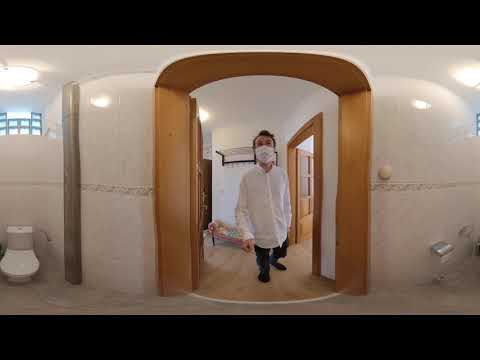In this grainy, slightly pixelated image, reminiscent of a video screenshot, we see a man with dark hair standing in the doorway of a bathroom within a home. He is dressed in a long-sleeve white button-up shirt, dark pants, and dark shoes, and he is wearing a white surgical mask. The bathroom features white walls with beige tile — highlighted by a decorative strip of tile midway up the wall — and a light brown floor. On the left side of the image, partially visible, is a white toilet beneath a barred window, with a toilet paper dispenser on the right of the toilet. Toward the center, there is a small pink floral bench with a coat rack above it, suggesting this area doubles as a small sitting or entrance area. The image's top and bottom have black borders, indicating it’s a screenshot, possibly from a low-quality camera.